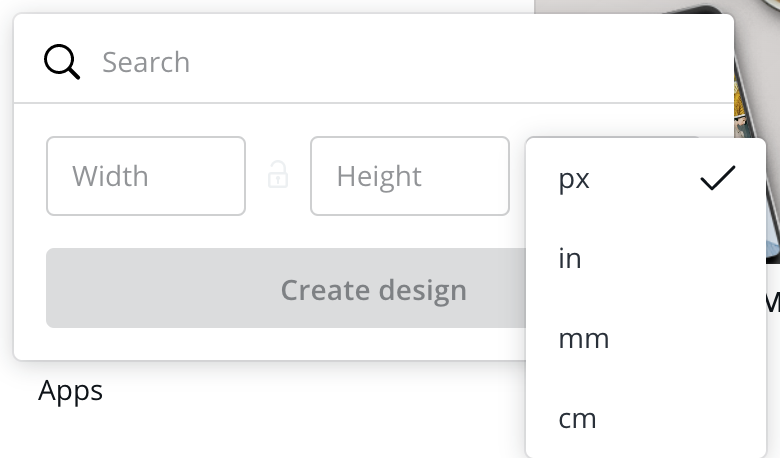The image is a screenshot featuring an empty search bar prominently displayed at the top. Below the search bar, there are fields labeled "Width" and "Height," accompanied by dropdown menus for specifying units of measurement such as pixels (PX), inches (IN), millimeters (MM), and centimeters (CM). Further down the interface, there's a conspicuous "Create Design" button. Additionally, the word "Apps" is visible beneath this button, indicating a navigation or option panel related to applications. The entire screenshot appears to capture only this specific section of a design interface.